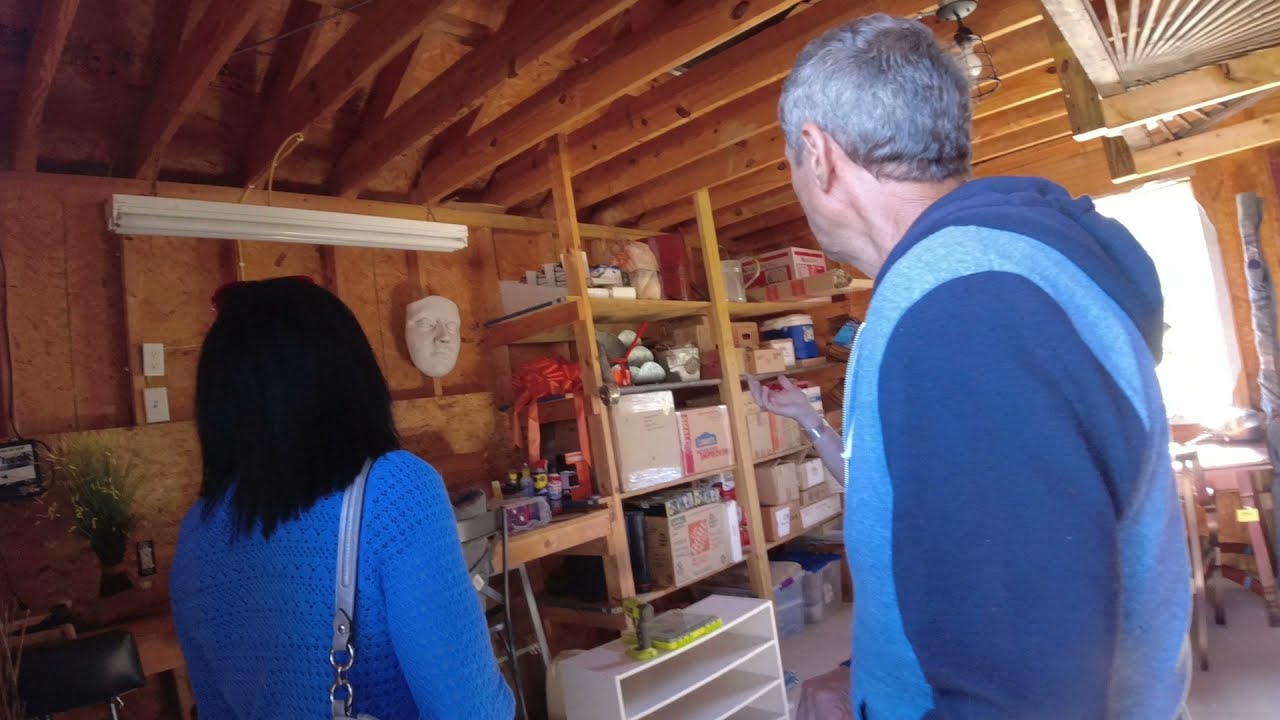In this image, we see the backs of two individuals standing inside an unfinished garage or storage room, which features exposed wooden rafters, uninsulated walls, and wooden shelves packed with various household items and cardboard boxes. The man on the right has gray hair and is wearing a light and dark blue sweatshirt. The woman on his left has shoulder-length dark brown hair, and she is dressed in a blue sweater with a gray purse strap over her shoulder. They appear to be conversing with another person, whose hand is partially visible in the frame. The shelves they are inspecting are filled with assorted belongings, including a ceramic Santa Claus, and a white mask of a face hanging on the wooden wall with a light fixture above it. In front of the shelves, there is a small white shelf with what seems to be a sponge on top of it. Near the shelves, a workbench is also visible, cluttered with additional items.